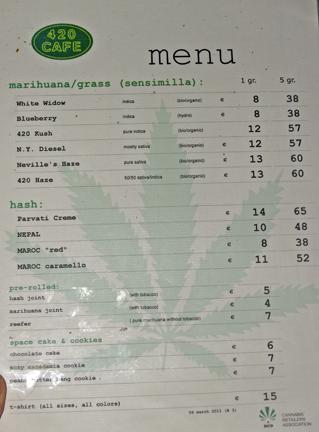The image showcases a detailed menu from a cafe named "420 Cafe," which appears to have a marijuana-themed focus. The cafe's name, "420 Cafe," is displayed prominently in light green text against a dark green background. The menu header has the word "Menu" in black lettering set against a muted white background, which gives it a slightly vintage appearance. 

In the background of the menu, there is a subtle illustration of a marijuana plant. The top section of the menu is labeled "Marijuana/Grass Sensimilia" and lists various strains available for purchase, including White Widow, Blueberry, 420 something, NT Diesel, Nivelles, Hayes, and 420 Maza. The menu specifies prices based on gram quantities, with options for both single grams and five grams.

Below the marijuana section, the menu offers a selection of hashish with four distinct varieties, again detailing prices for one gram and five grams. Further down, though the text becomes difficult to read, it appears that the menu also includes items like space cakes and cookies, which are sold by the gram.

The overall design of the menu is kept simple and functional, with black text on a light background, enhancing readability without the use of vibrant colors.